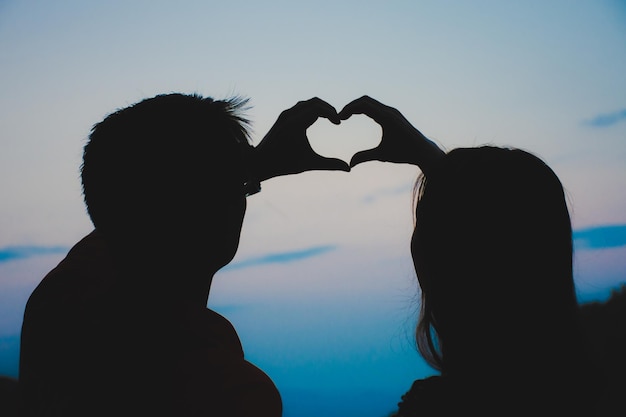In this photograph, the silhouette of a couple is perfectly captured in a romantic scene against a gradient sky of light blue and light purple hues. The man on the left raises his left arm, his fingers forming the curve of a 'C.' The woman on the right lifts her right hand, creating a mirrored 'C' with her fingers. Together, their hands form a heart shape, symbolizing their deep love and connection. The detailed shadows of their forms are set against the softly lit sky, enhancing the intimacy and tenderness of the moment.